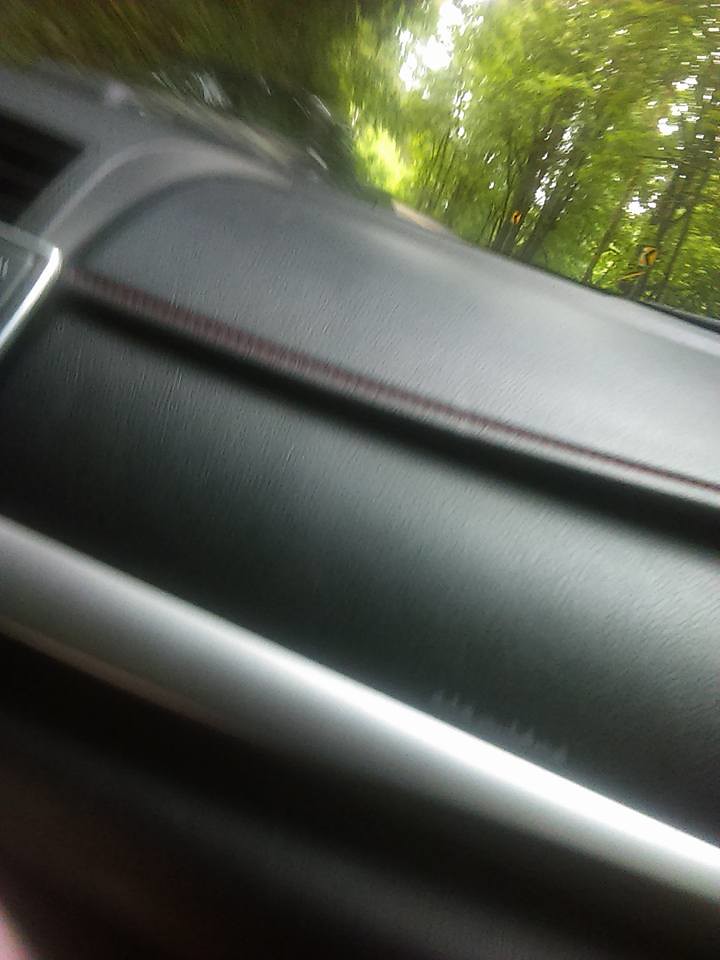The photograph, taken in portrait format and in color, captures a detailed interior view of a vehicle from the front passenger seat at a diagonal angle. The sleek, black leather interior dominates about 80% of the image, showcasing a luxurious dashboard and lower compartment where a passenger's legs would rest. A distinctive white metal pole, likely the door handle, is prominently visible. The gray dashboard features a small plastic strip running across it, though some wording present is blurry and indiscernible. The upper portion, approximately 20% of the photo, reveals a scenic view through the windshield. The narrow road outside is enveloped by dense greenery, with large trees displaying mossy light green leaves and dark brown branches. Bright sunlight filters through the treetops, particularly noticeable in the top right corner, enhancing the vibrant outdoor scene.